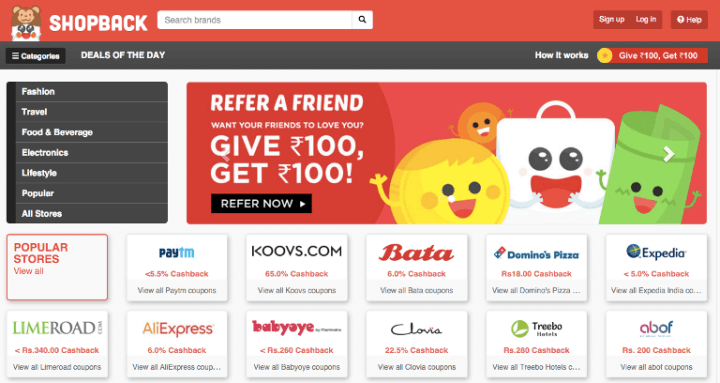The image showcases the homepage of the ShopBack website. Dominating the top-left corner is the ShopBack logo, accompanied by an animated character resembling a monkey. The upper background is predominantly red, creating a vibrant and eye-catching header. Adjacent to the logo, a white search bar spans across the top. On the far right, the navigation options include 'Sign Up,' 'Log In,' and 'Help.'

Below this red header, the background transitions to black, highlighting key sections: 'Categories' on the left and 'Deals of the Day' in white text. Further right, there's 'How it Works' and a striking red section promoting "Give $100, Get $100," accentuated by a yellow circle.

The main content area is primarily white, with various categories listed on the left, such as Fashion, Travel, Food & Beverage, Electronics, Lifestyle, Popular, and All Stories. On the right, the background shifts to a darker red, featuring a referral promotion that reads, "Refer a friend, want your friends to love you? Give $100, Get $100. Refer Now," with a black rectangular button. Accompanying this promotion are four animated, smiling objects in yellow, orange, white, and green.

Below the referral section are twelve square icons representing popular websites and companies, presumably partners of ShopBack, all set against a white backdrop.